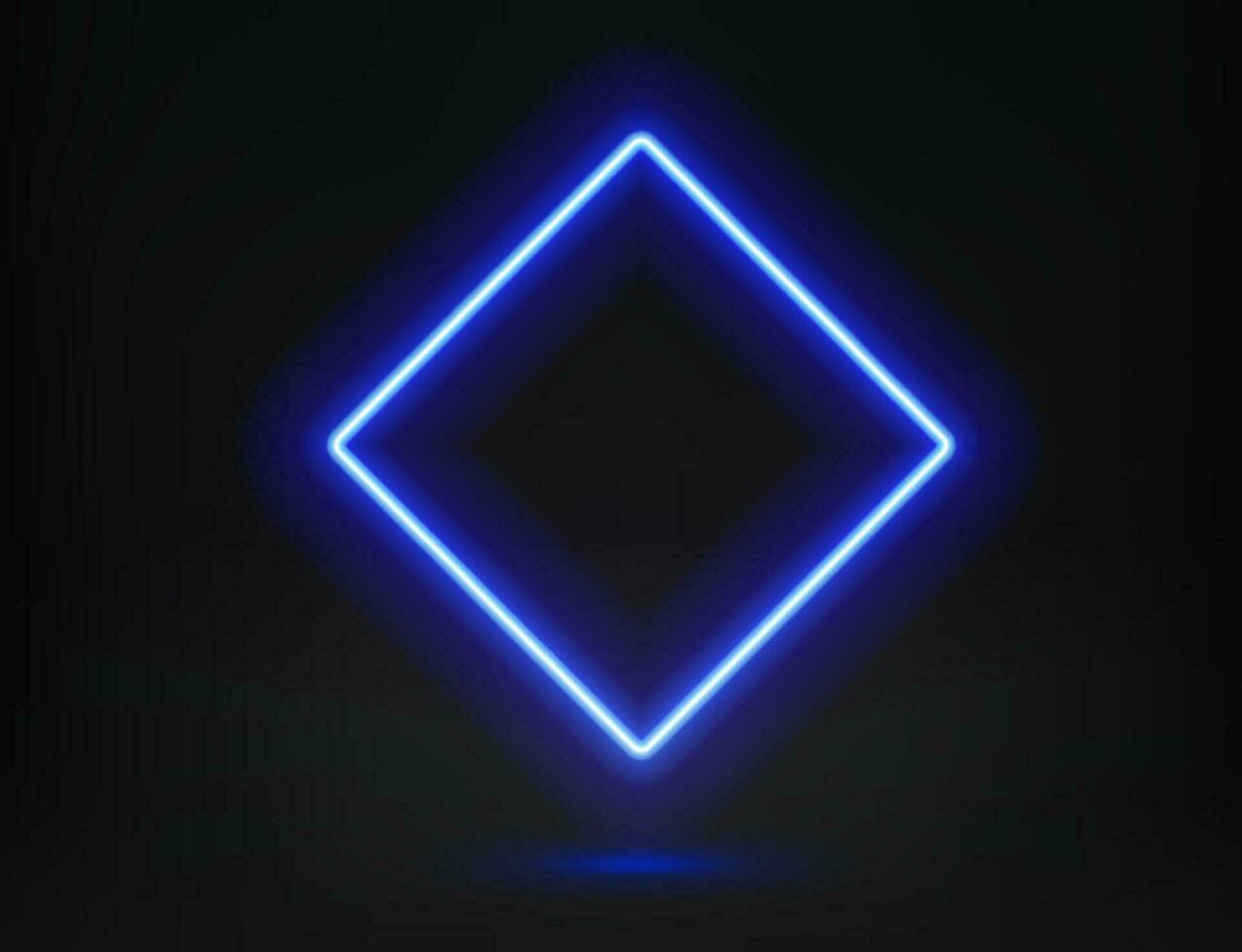The image portrays a striking visual of a neon-lit square set against an all-black background. This square is tilted on its side to create a diamond shape, generating a compelling almost three-dimensional effect. The diamond emits a neon royal blue hue with a white inner border that seems illuminated. Notably, there is a darker blue square at its core, adding to the depth perception of the light. Subtle hints of green and wavy lines can be discerned in the predominantly black background, which amplify the contrast and mood of the image. Additionally, a faint blue shimmer is visible beneath the diamond, creating an illusion of a shadow or reflection. This captivating geometric artwork emphasizes the stark contrast between the glowing diamond and the enveloping darkness.